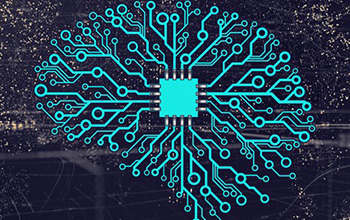The image is a horizontal rectangle, approximately one and a half times as wide as it is tall, featuring a striking close-up of a light blue computer chip at its center. This chip, resembling a microchip from a circuit board, is adorned with four little metal projections on each of its four sides, making a total of 16 connections. Each metal piece transitions into light blue wires that branch out into intricate patterns forming the shape of a human brain when viewed from the side. These branching wires contain circular nodes, mimicking the neural network of a brain and creating a complex, web-like structure. The background of the image is predominantly black, scattered with numerous small yellow or orange dots that resemble stars, alongside some faint gray lines. This detailed backdrop adds depth to the digital representation, giving it a cosmic, star-studded appearance.